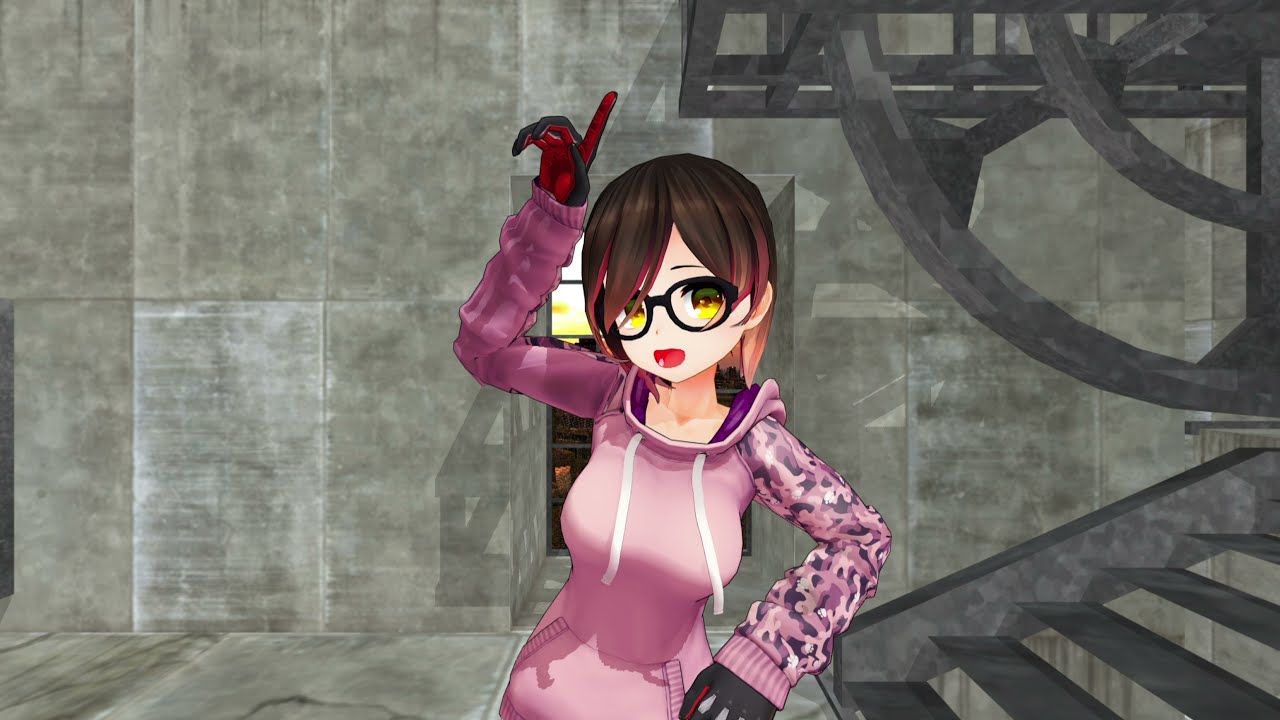This anime avatar is a young woman with short, shoulder-length hair featuring a dark brown to pink gradient ombre, fading into pink tips. She is wearing a bright pink hoodie with white drawstrings hanging in front of her chest. The hoodie has distinct sleeves: the left sleeve is dark purple, while the right sleeve has a pink, purple, and gray camouflage pattern. She sports black-rimmed glasses with clear lenses, revealing her eyes which appear to have yellow and brown tints. Her lips are adorned with vibrant red lipstick. She is wearing gloves that are black on the top and red on the palms. The avatar is pointing up to the top center of the image with her right index finger, striking a pose reminiscent of disco dancing. Positioned in a concrete room with tall ceilings, a window is visible in the background, alongside a gray staircase located in the bottom right corner of the image. Additionally, in the top right corner, there are two curved objects attached to a balcony or railing.